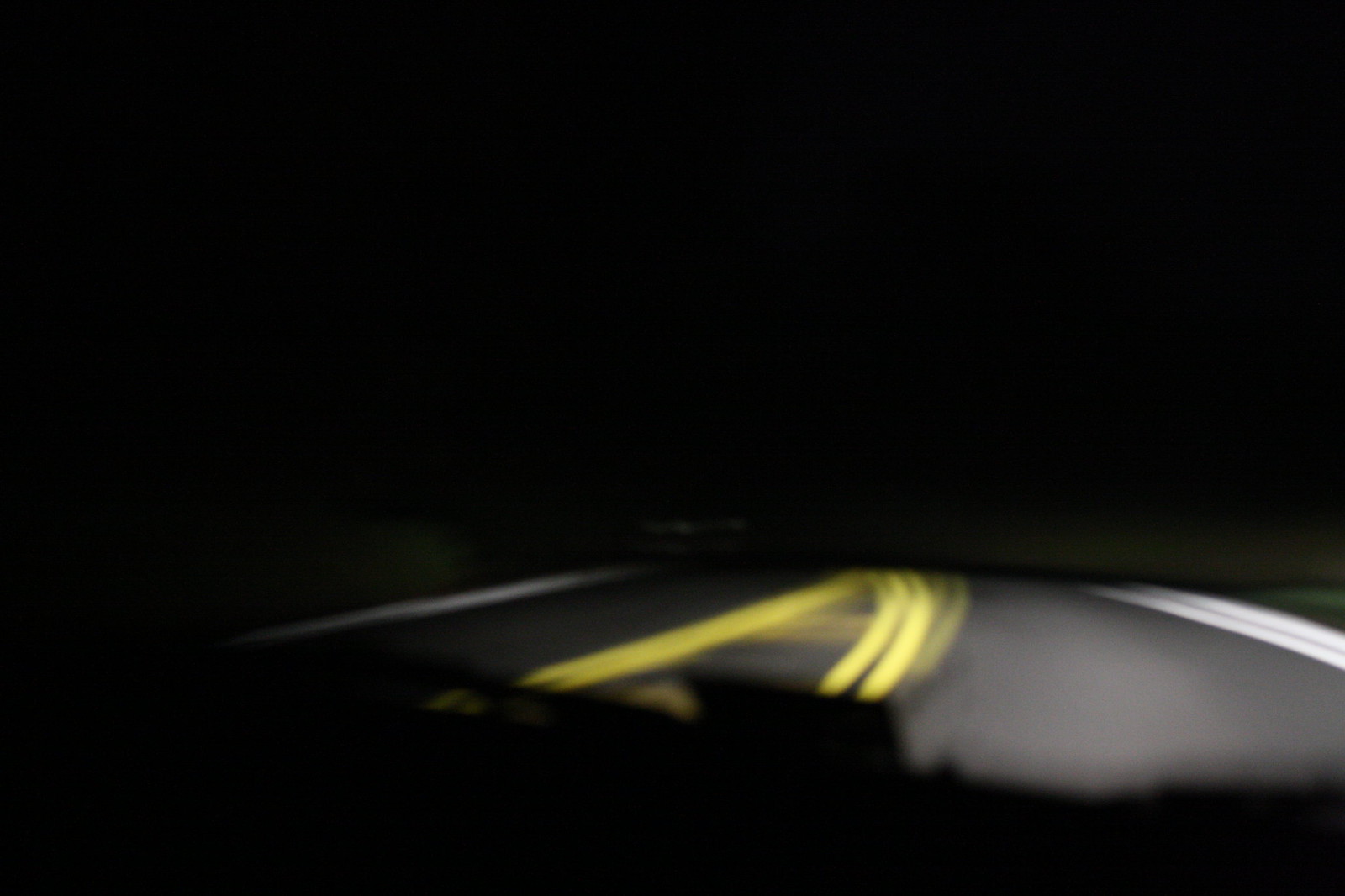This is an extremely blurry nighttime photograph taken from inside a car, looking out onto a roadway. The background is pitch black, with a faint, lighter color at the horizon just above the road. The roadway stretches off into the distance with blurry yellow lines running down its center and white lines on either side, all set against a gray road surface. Dominating the lower portion of the image is a dark shape identified as the car's dashboard, which extends from the center left to the lower right. A prominent, blurred yellow line, possibly a reflection or light, runs across this dark foreground shape, looping up and curling around. Despite these details, the overall image remains abstract and unfocused, contributing to its mysterious and indistinct quality.